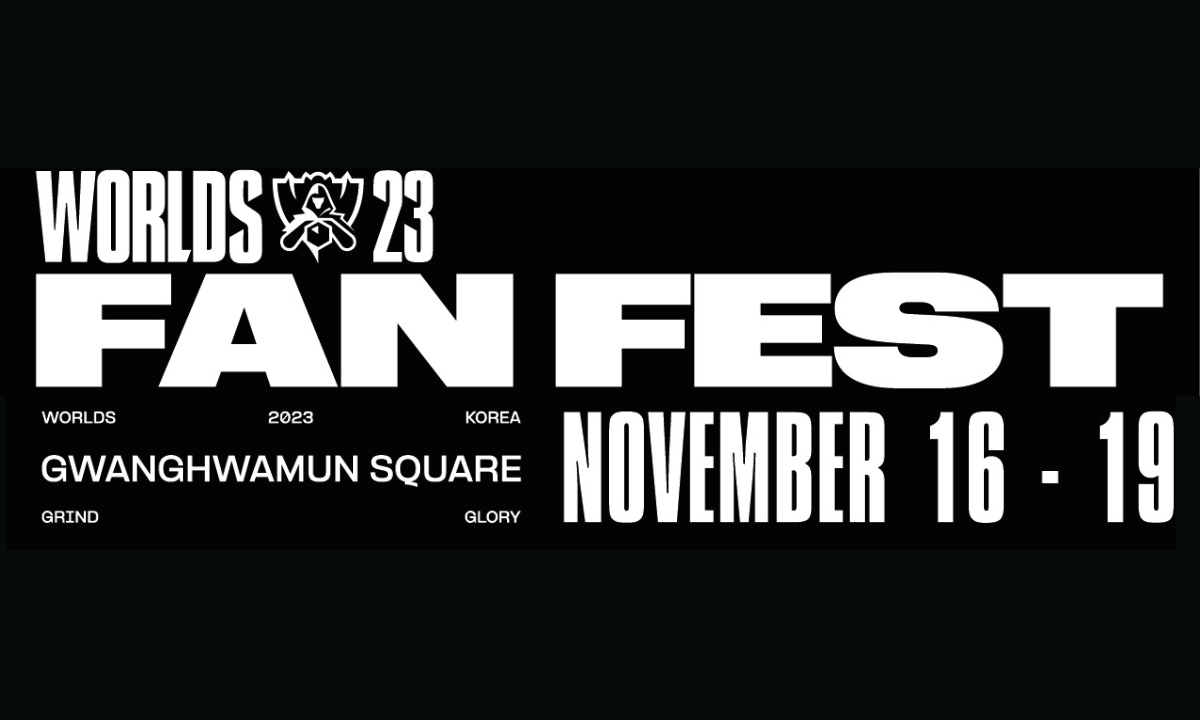The poster presents a stark black background dominated by bold white text and a central emblem. At the top, the text "WORLDS" is accompanied by a logo depicting a hooded figure with a hexagon in front, suggesting the League of Legends event, followed by "23" for the year 2023. Below, in striking capital letters spanning the width of the image, it reads "FANFEST." Underneath this, additional details are layered in smaller white text: "WORLDS 2023" and "Korea." The location is specified as "Gwanghwamun Square," emphasizing the venue's prominence. The dates "November 16-19" are prominently displayed, indicating the event duration. At the very bottom, in small text, the words "GRIND" and "GLORY" are juxtaposed, adding a motivational flair. This concise, impactful layout makes it versatile for use as a poster, bumper sticker, or various forms of advertisement.